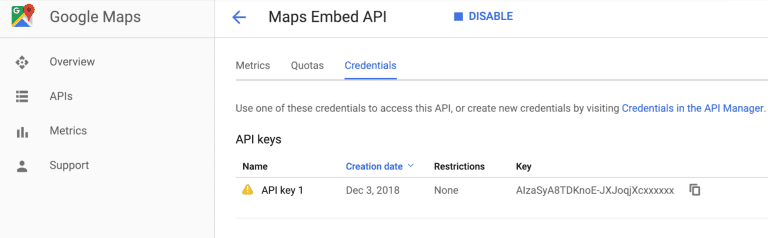This image captures a detailed view of the Google Maps interface, specifically focused on the API management section. 

On the left side of the screen, a Google Maps listing is displayed with options labeled "Overview," "APIs," "Metrics," and "Support" situated below the listing. The right side prominently features the "Maps Embedded API" section, which allows the user to enable or disable the API. Below this, options labeled "Metrics," "Quotas," and "Credentials" are displayed.

A highlighted section provides instructions, stating, "Use one of these credentials to access the API or create new credentials by visiting Credentials and the API Manager.” The terms "Credentials" and "API Manager" are highlighted in blue, indicating clickable links to respective portals.

Additionally, the image shows API keys listed, including one created on December 3, 2018. The listing mentions that there are no restrictions associated with this key. The actual API key is displayed as "A1zaSYA8TDKNOE-JXJOQJXCXXXXX." Next to the key, there is an option to click and copy the key for later use.